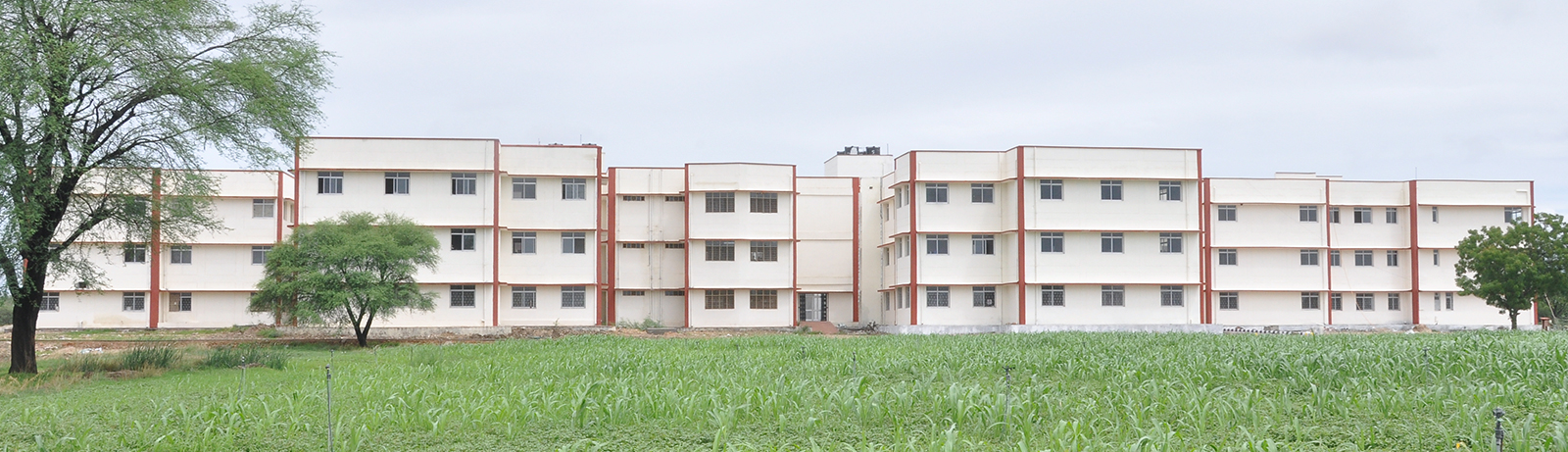The image depicts a residential complex, potentially apartments, dormitories, or condos, consisting of a series of interconnected buildings each three to four stories tall. The buildings are predominantly white or cream with distinctive brown-orange trim along the edges, contributing to their boxy, flat appearance. Each level has rows of rectangular windows with plain, white panes, totaling three windows per side per unit. In the foreground stretches a slightly overgrown grassy field, sprinkled with three trees—two on the left and one on the right. The lush green leaves on the trees contrast with the overcast sky above, which appears grayish with a hint of blue. The scene exudes a suburban tranquility despite the somewhat neglected lawn in need of mowing.